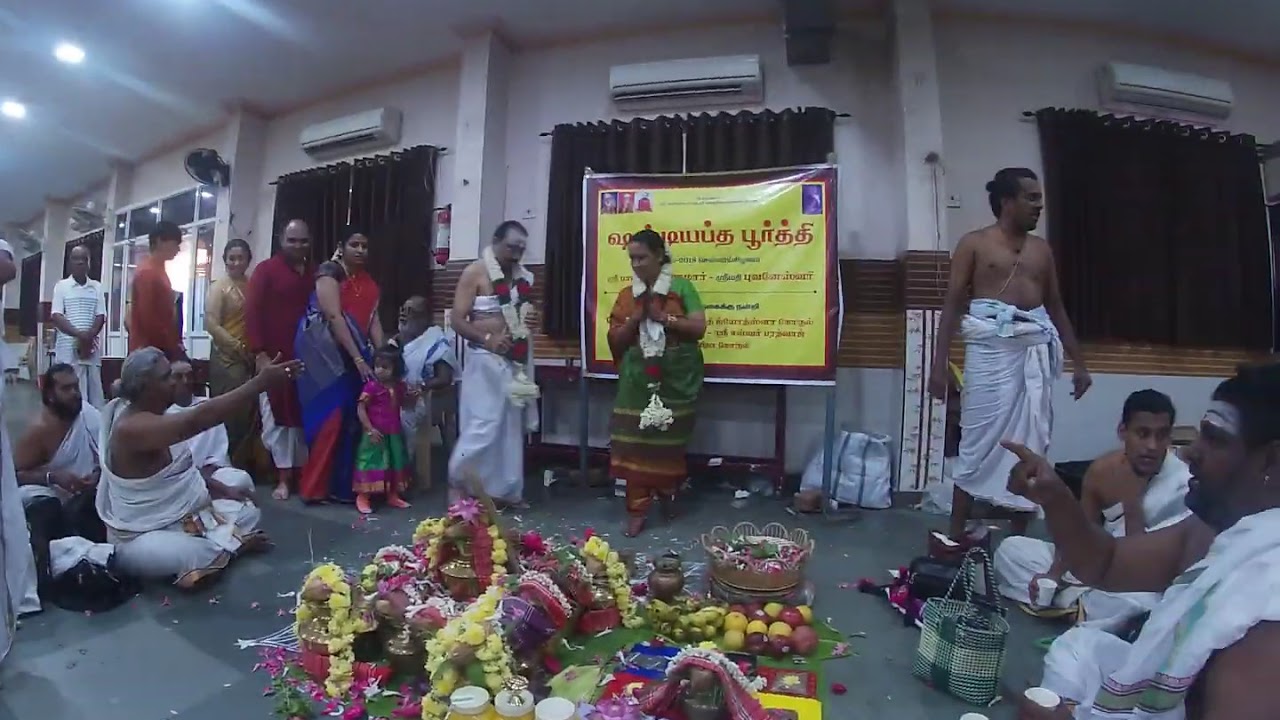The photograph captures a vibrant and culturally rich scene, likely from an Indian or Sri Lankan festival or religious gathering. At the center of the image, a blanket is laid out, adorned with an array of colorful decorations, fruits, flowers, and possibly strands of confetti, signifying a festive or religious offering. 

Prominently in the middle stands a woman dressed in a green dress with her hands clasped in a praying pose, symbolically representing reverence. Beside her is a man in a white sash, both of them adorned in what appears to be traditional religious paraphernalia draped around their shoulders. Behind this central pair is a diverse group of individuals, some of whom are wearing traditional and colorful Indian attire, while others don white robes.

To the left of the main group is a cluster of individuals dressed in white robes, sitting down. On the right, several people in white robes gather, with one person seated and pointing towards some of the individuals across the room, another standing and looking upwards. A family group dressed in red, blue, pink, and green can be seen, with an older gentleman in white seated beside them. They all seem to be part of this vibrant gathering, likely inside an indoor setting, as indicated by the walls and a sign in a different language visible in the background.

The scene is lively and communal, rich with tradition and festivity, encapsulating the essence of a cultural celebration centered around offerings of food and flowers.